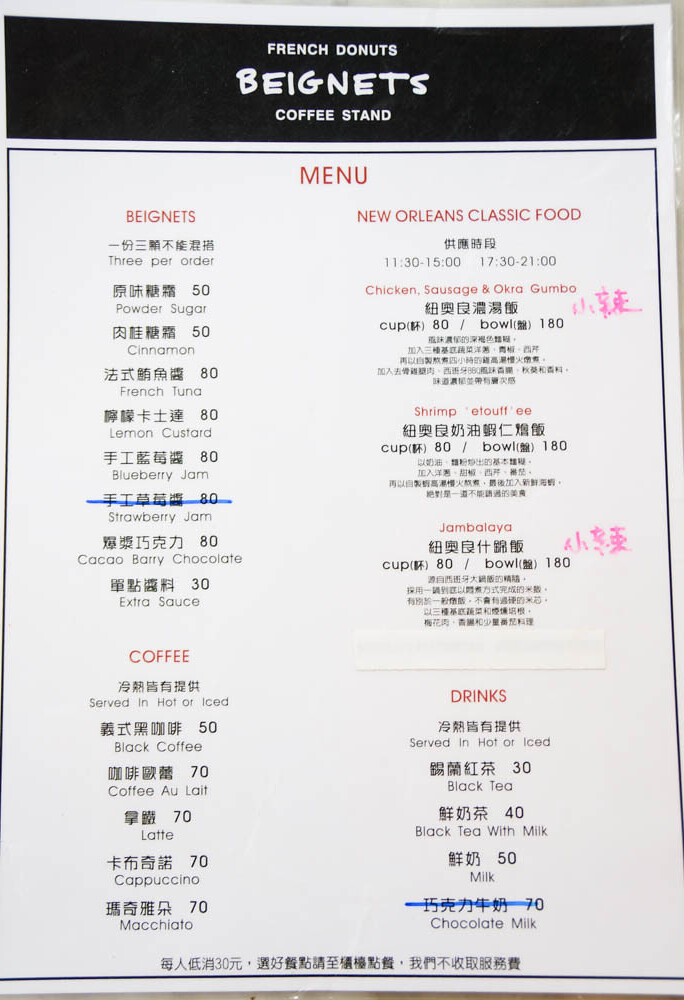This photograph captures a detailed menu printed on elongated white paper. At the very top of the menu, a prominent black banner displays the words "French Donuts" with "B-E-I-G-N-E-T-S" spelled out just below it. Directly underneath, "Coffee Stand" is inscribed, setting the theme for the offerings.

Moving down to the main section of the menu on a white background, the word "Menu" is boldly printed in red ink. Below this header, the items are listed in both English and what appears to be Chinese.

On the right side of the menu, a headline in red print declares "New Orleans Classic Food." Under this heading, various traditional dishes are enumerated. The first dish listed is "Chicken Sausage and Okra Gumbo," followed by its name written in Chinese. Next is "Shrimp Etouffee," again with the corresponding Chinese characters beneath. The same format is used for "Jambalaya," where the name appears in red ink with Chinese letters below.

The menu also highlights "B-E-I-G-N-E-T-S" available in various flavors. Additionally, it mentions "Coffee" with the corresponding foreign language script. The drinks section follows the same bilingual format, ensuring clarity and accessibility for a diverse audience.